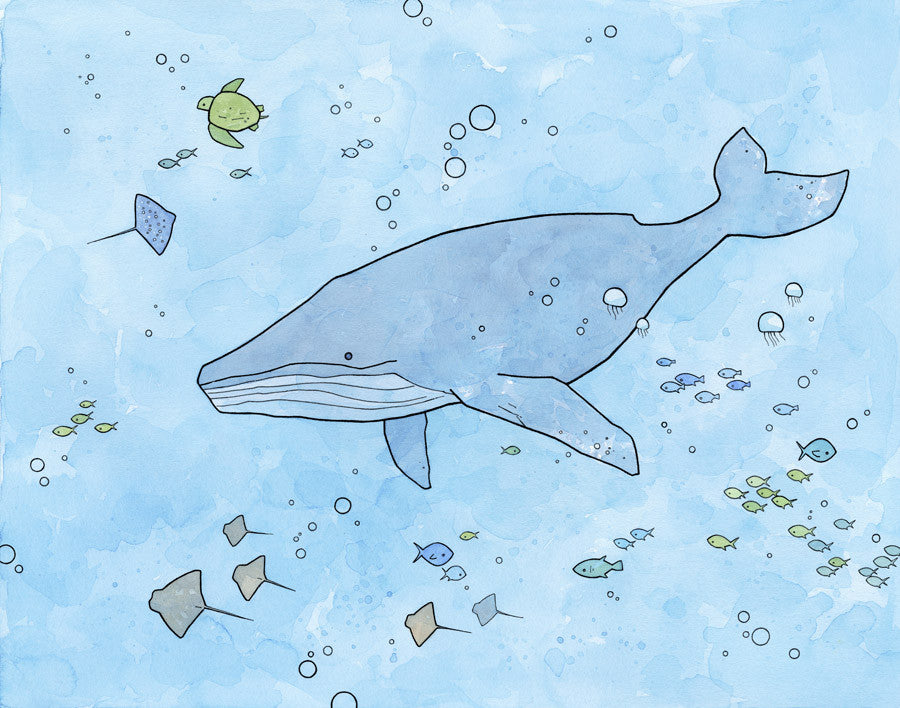The illustration is a watercolor depiction of an underwater scene, featuring a variety of marine life. Dominating the center is a large beluga whale, light blue with a lighter underbelly, gracefully swimming amidst the ocean blue hues. Surrounding the whale, the scene is accentuated by intricate black ink outlines. The background blends shades of light and dark blue with occasional splotches, creating a translucent effect that lets the blues permeate through the figures. On the upper left, a green sea turtle swims serenely with several smaller fish, while on the bottom right, schools of tiny green and blue fish dart around with lively bubbles interspersed, indicating their animated existence. Jellyfish linger on the right side, their delicate forms adding to the tranquility of the scene. The illustration also includes a variety of rays: a single blue ray glides above the whale, and beneath it, a group of beige rays. Every element — from the fish to the sea turtles, stingrays, jellyfish, and the majestic whale — exudes a sense of contentment and harmony within this underwater paradise.